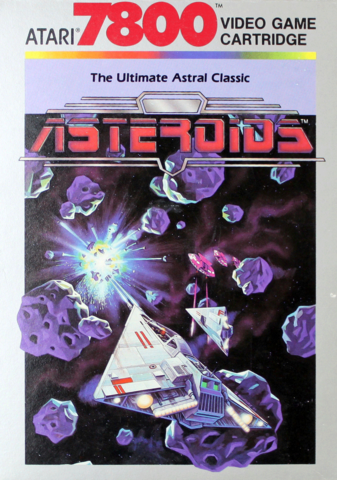The image showcases the front of a vintage Atari 7800 video game cartridge titled "The Ultimate Astro Classic." Dominating the top portion, the text "Atari 7800" appears, with "Atari" in black and "7800" in bold red lettering. The phrase "video game cartridge" accompanies it. Below this header, a silver banner highlights the game's title: "Astro" in red and black.

Prominently featured in the center of the image is a dynamic cartoon illustration set against a black starry space backdrop. In the scene, a white, triangle-shaped spaceship adorned with red accents and emitting white lights from its rear is actively engaged in an asteroid battle. A blue laser beam emanates from the spaceship, striking a purple asteroid, creating a dramatic explosion with shards of debris scattering in various directions.

Additionally, a secondary, smaller spaceship appears to the right of the main one, also navigating through the asteroid field, which includes some pink-hued asteroids. The entire composition conveys a sense of action and vintage sci-fi excitement typical of classic space shooter games.